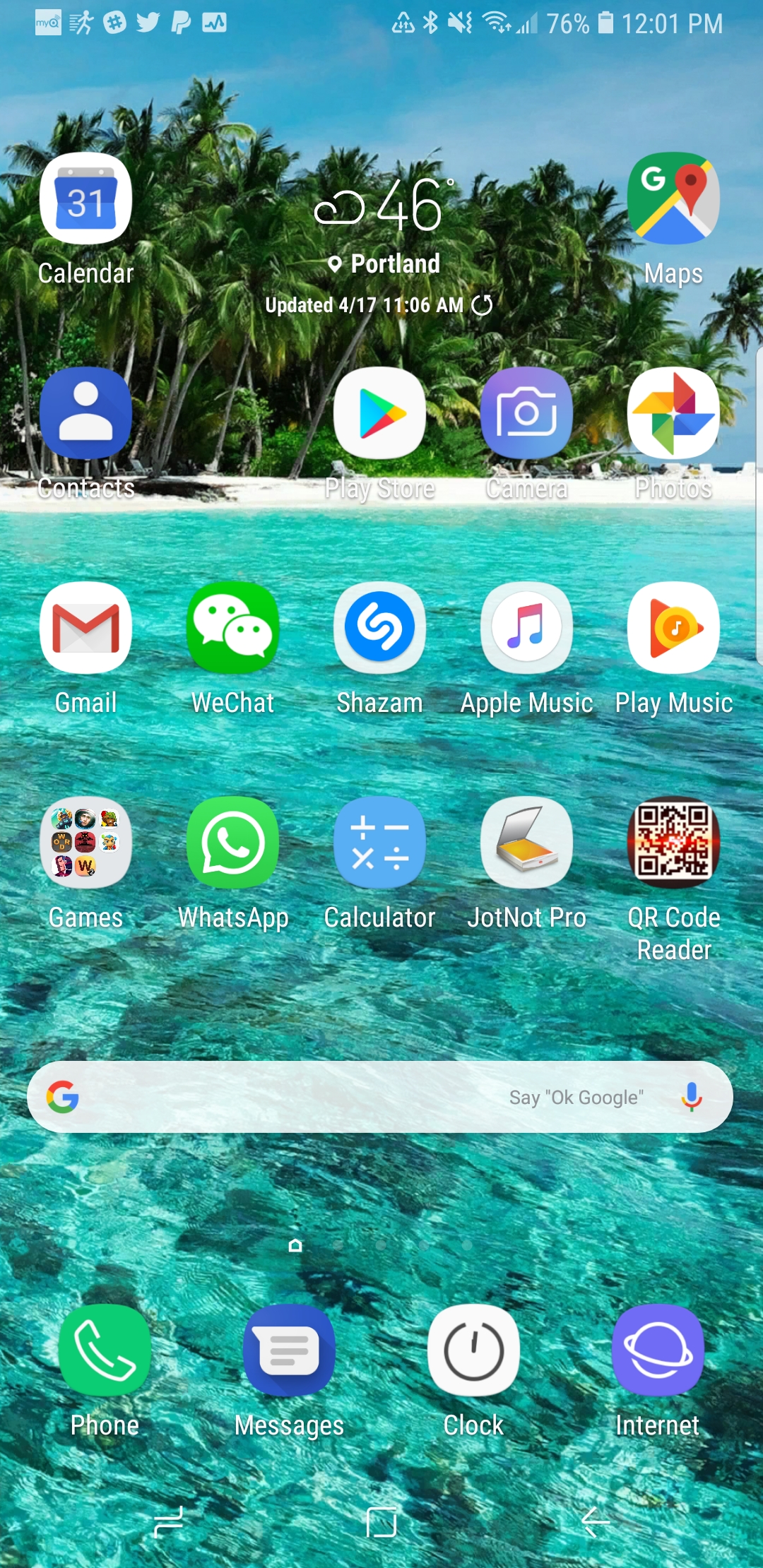Here is a detailed and cleaned-up caption for the image described:

---

The image showcases an Android smartphone with a vibrant beach-themed wallpaper, featuring crystal clear water and lush green trees in the background. At the top left of the screen, there's a status bar displaying several symbols: a square with text inside, dashes, a circle with a hash mark, a photo symbol, a PayPal icon, a white square with a squiggle, a triangle, a dashed triangle, the Bluetooth logo, a muted speaker icon, a Wi-Fi symbol indicating active data transfer, a battery icon filled to 76%, and the time reading 12:01 p.m.

The home screen is populated with numerous app icons neatly arranged. Starting from the top left:
- Calendar (a white square with "31" in it)
- Maps (a map pin symbol)
- Contacts (a blue square with a white person icon)
- Play Store (a multicolored triangle: blue, yellow, red)
- Camera (a camera icon)
- Photos (a photo symbol)
- Gmail (an envelope in white and red)
- WeChat (a green square with two speech bubbles containing dots)
- Shazam (a blue circle with an "S" in the center)
- Apple Music (a musical note icon with a blue-to-red gradient)
- Play Music (an orange triangle with a circle and musical note)
- A folder labeled "Games" filled with various game icons
- WhatsApp (a green square with a phone bubble icon)

Additionally, there are utilities like:
- Calculator (grid with symbols for addition, subtraction, multiplication, and division)
- Dot Not Pro (an icon suggesting an open scanner with an orange surface and reflective screen)
- QR Code Cleaner (a QR code reader symbol)

At the bottom of the screen, a white search bar with rounded edges and a microphone icon displays the text "Say, 'OK Google'". The dock at the bottom of the screen includes:
- Phone app (green square with a phone symbol)
- Messages (a blue bubble with a white chat bubble inside)
- Clock
- Power icon
- Internet browser